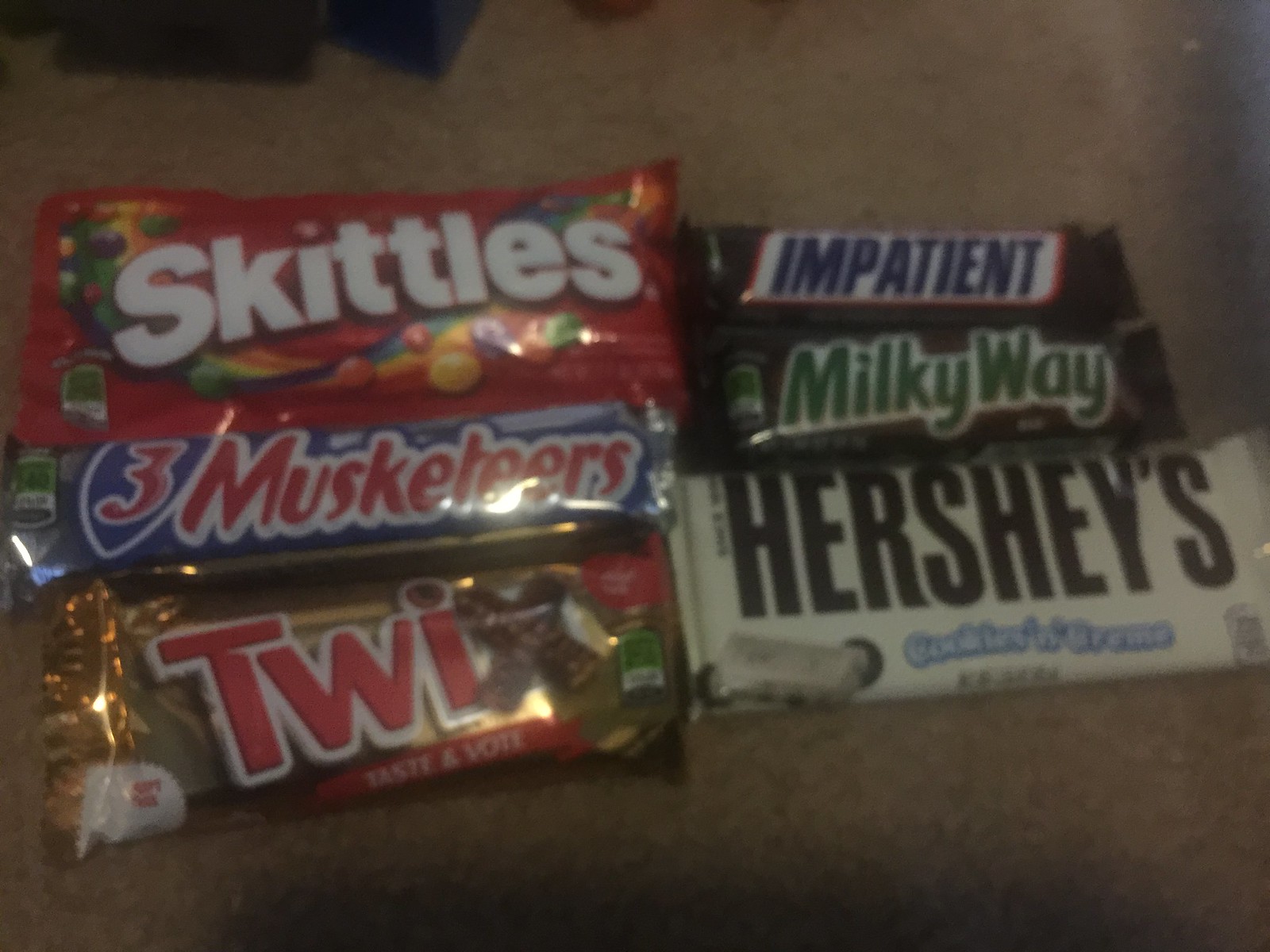In this image, there are six king-sized candy bars arranged on a light brown or gray carpeted floor. The candy bars are displayed in two columns, each with three candy bars. Starting from the top left, there is a red Skittles package with white text and rainbow-colored Skittles illustrations. Below the Skittles is a Three Musketeers bar, featuring a gray wrapper with red, white, and blue text. Directly below that is a Twix bar in gold packaging with red text. On the top right, there is a Snickers bar, but instead of "Snickers," it says "Impatient" in blue text on a white background with a red border. Below the Snickers, we find a Milky Way bar, which has a brown wrapper and green text. Lastly, at the bottom right, there is a Hershey's Cookies and Cream bar, which has a white wrapper, dark brown "Hershey's" text, and blue "Cookies and Cream" text. The image is slightly blurred, suggesting it was taken with a camera or phone that might have had a dirty lens.